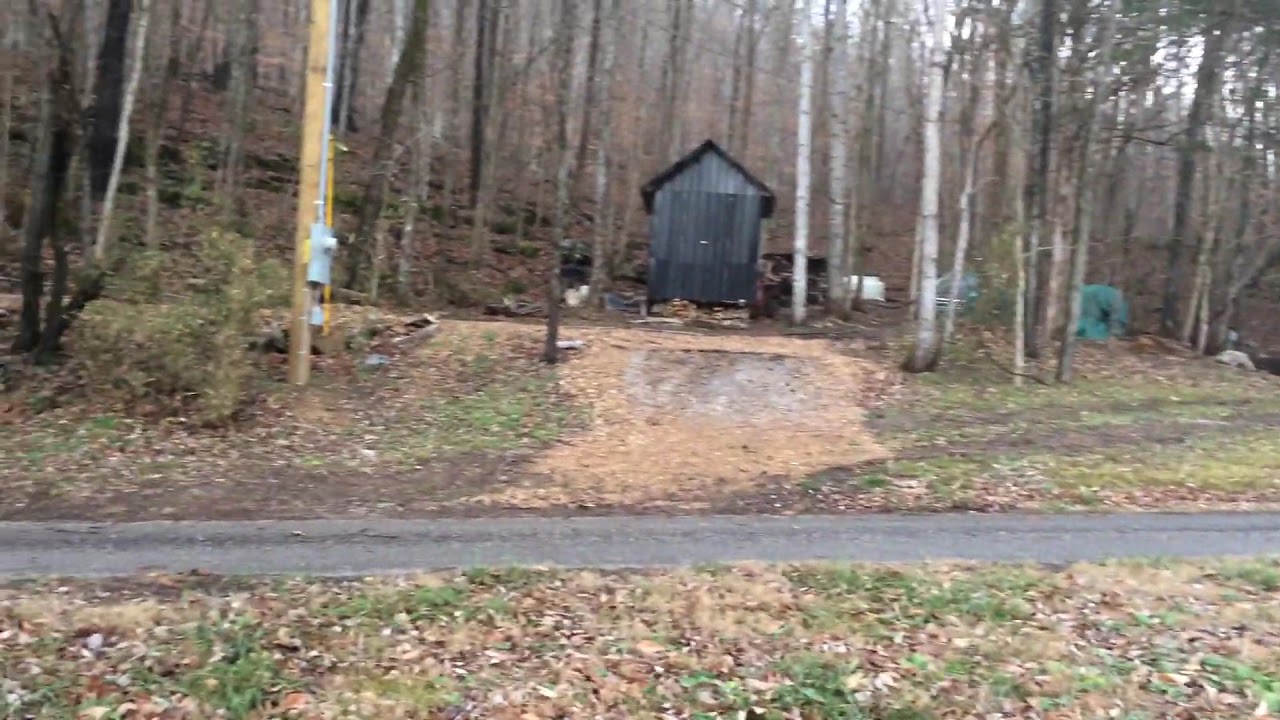In this somewhat blurry and slightly tilted photograph, taken on a cloudy day, we see a dark gray or black shed, constructed from corrugated metal sheets, standing amid tall and skinny trees that resemble birch, with their slender trunks and sparse branches. These trees suggest a wintry or autumnal setting, as their tops are out of frame and their branches lack dense foliage. The grass surrounding the shed appears patchy, partially green but mostly covered with fallen leaves. To the left of the shed, near a narrow, curved, or short driveway, there is a utility pole with some sort of meter attached, as well as a tiny mailbox. There seem to be various miscellaneous items typically found around a shed scattered about, contributing to the rural feel of the scene.